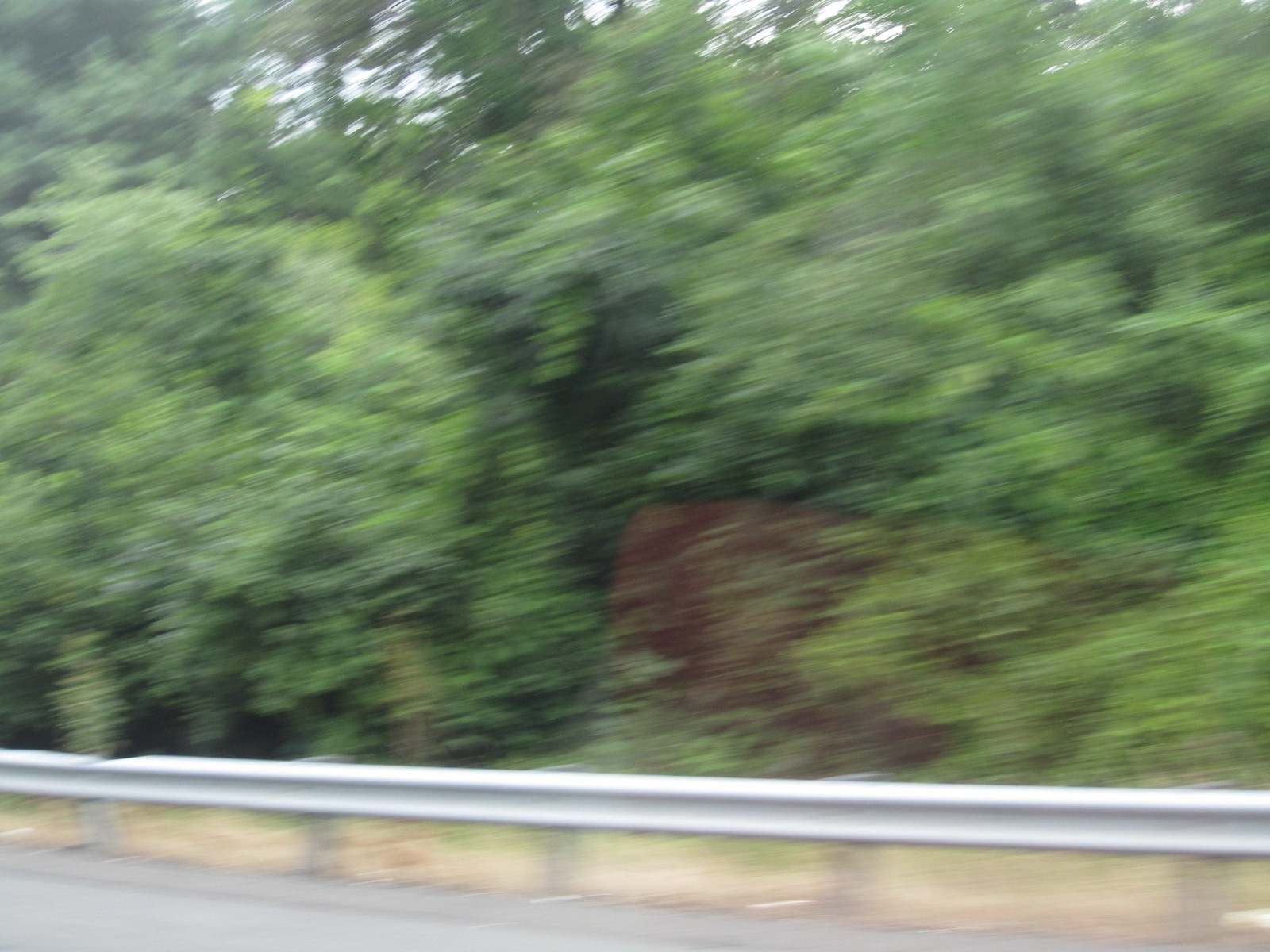This is a very blurry image taken from inside a moving car, capturing the view outside the window. The scene features a dense forested area with thick greenery, abundant branches, and leaves. At the top of the photo, patches of blue sky and sunlight are visible through the foliage. The bottom of the image shows a silver guardrail running the length of the picture, supported by metal posts embedded in the ground. A small portion of a regular asphalt road starts at the bottom left corner. Adding to the blur, a red reflection from inside the car is visible in the center of the photo. The overall impression is a quickly snapped shot while driving, where specific details and individual elements are hard to distinguish due to the significant blurriness.